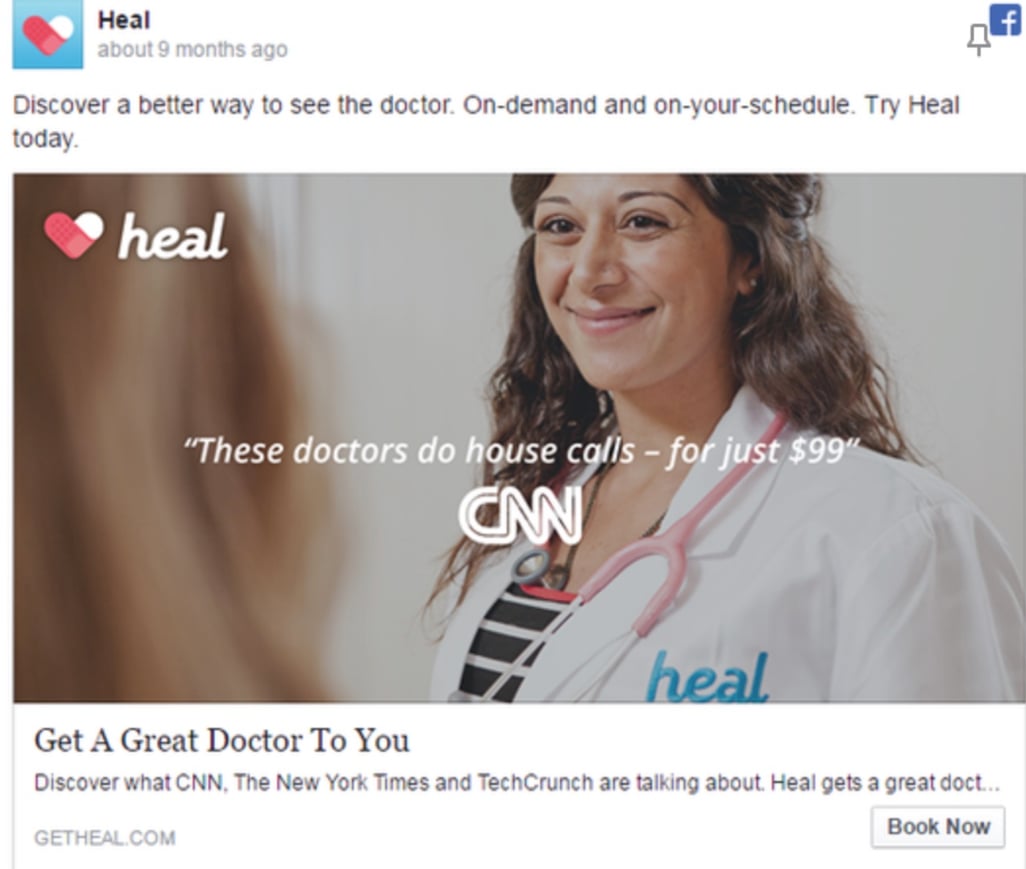The image depicts the homepage of a website called "Hale." In the top-left corner, the Hale logo, which consists of a small heart icon, is prominently displayed next to the site's name. The webpage indicates it was posted nine months ago. On the top right, there is a link to Facebook and a pin icon, allowing users to pin the website.

Beneath the main logo is an explanatory tagline: "Discover a better way to see the doctor on demand and on your schedule. Try Hale today." Below this tagline is a rectangular image featuring a smiling nurse, with the Hale logo also appearing in the top-left corner of the image. Centered within the picture, white text reads: "These doctors do house calls for just $99," attributed to CNN.

Under the image, there is a white panel containing black text that states: "Get a great doctor to you. Discover what CNN, the New York Times, and TechCrunch are talking about." At the panel's bottom-right corner is a white button featuring black text that says "Book Now," enabling users to schedule an appointment with a doctor on demand or according to their own schedule via the website.